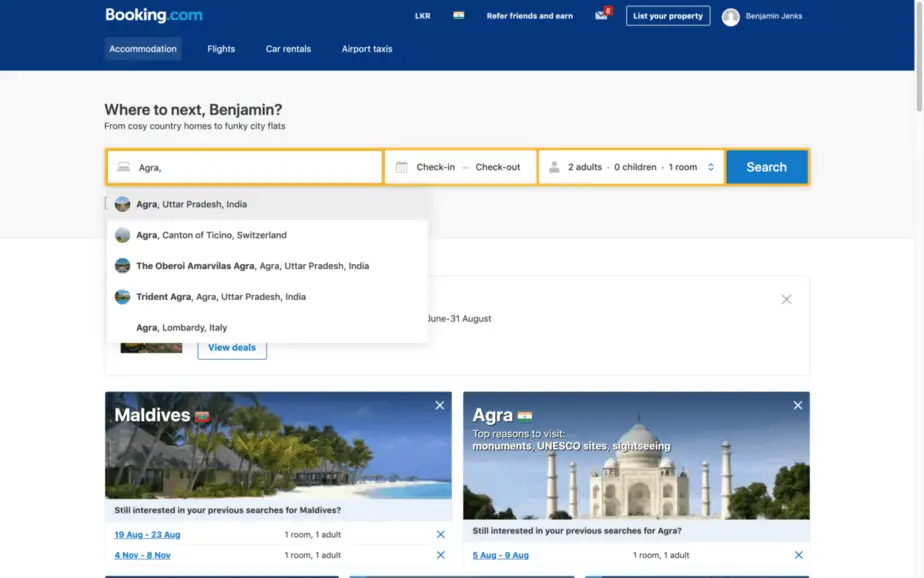This image is a screenshot taken from the Booking.com website. At the top of the screen, there's a dark royal blue banner with white text displaying the site's name, "Booking," and " .com" in a slightly lighter shade of blue. Within this banner, there are various clickable options such as "Accommodation," "Flights," "Car Rentals," and "Airport Taxis." Additionally, the top section features the currency displayed as "LKR," an option to "Refer friends and earn," an email notification icon showing the number eight, and links to "List your property" and the user's profile named "Benjamin Jenks."

Below the banner, the main section prominently features a search bar with placeholders like "Search destinations, properties, etc." Already filled are the search keywords "Agra," along with filters for "Check-in" and "Check-out" dates, "two adults," "zero children," and "one room."

Towards the bottom of the screenshot, there is a promotional section addressing the user, "Where to next, Benjamin?" followed by the tagline, "From cozy country homes to funky city flats." This section also displays thumbnail images of popular destinations, specifically the Maldives and Agra, offering a glimpse of some travel inspirations.